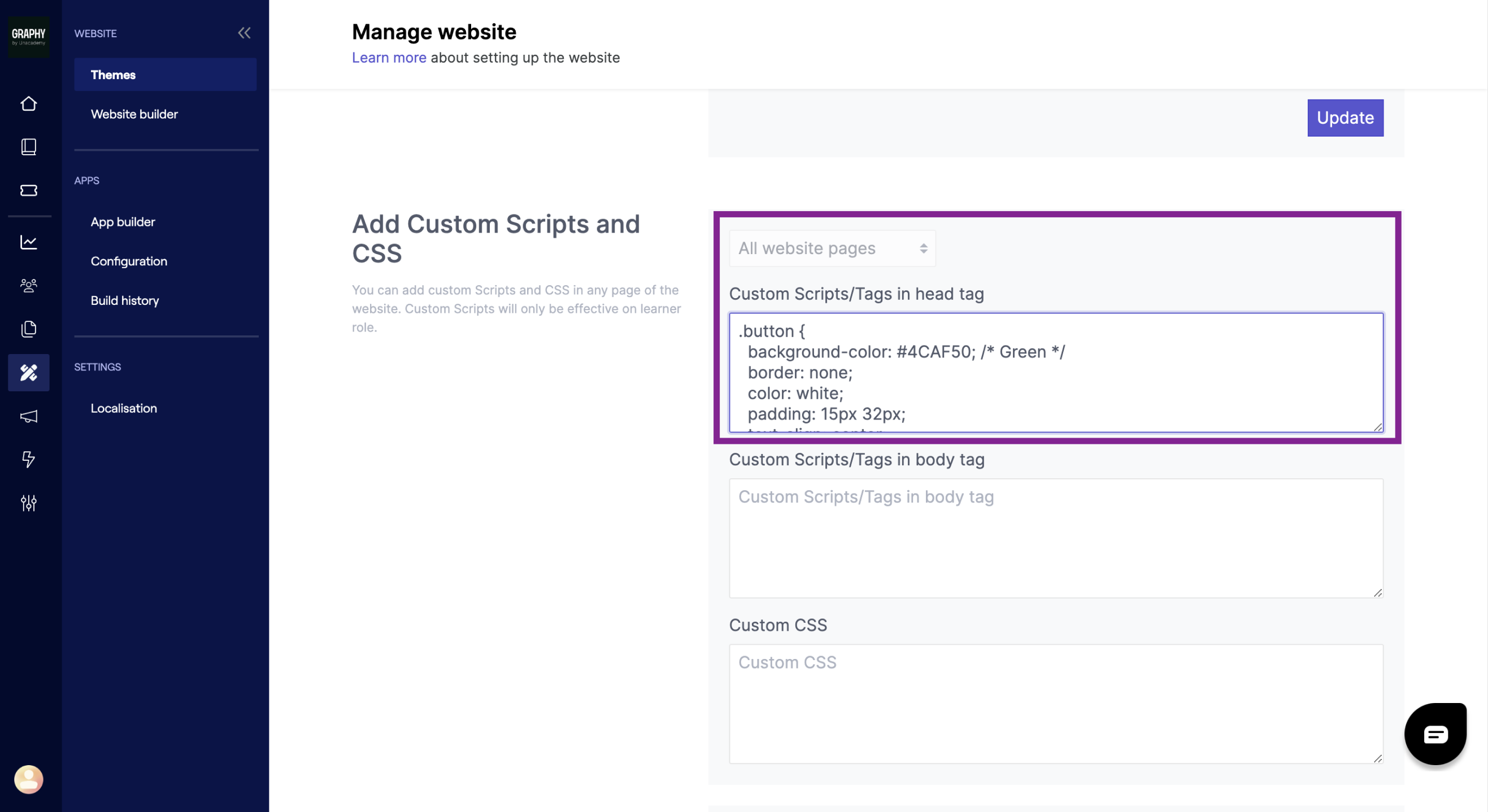This image is a screenshot from a web development platform, showcasing its interface. In the upper left corner, there's a blurry logo that appears to say "Graphy." Running down the left side of the interface are several unlabeled buttons represented by symbols. The currently active button, indicated as pressed, features an overlapping pencil and eraser icon.

On the right side of the interface, a tab has expanded to display various sections. At the very top, there's a section titled "Website Themes" and "Website Builder", followed by another section labeled "Apps," which includes options like "App Builder," "Configuration," and "Build History." The last section visible is "Settings," with a sub-option for "Localization."

Dominating the center of the screenshot is a prominent header that reads "Manage Website," accompanied by a subtext offering guidance on setting up the website. Below this, there is a section titled "Add Custom Scripts and CSS."

To the right, there is an outlined purple rectangle marked "Custom Scripts / Tags" and "Head Tag." Within this rectangle is a text box containing numerous lines of custom website scripting written by the user.